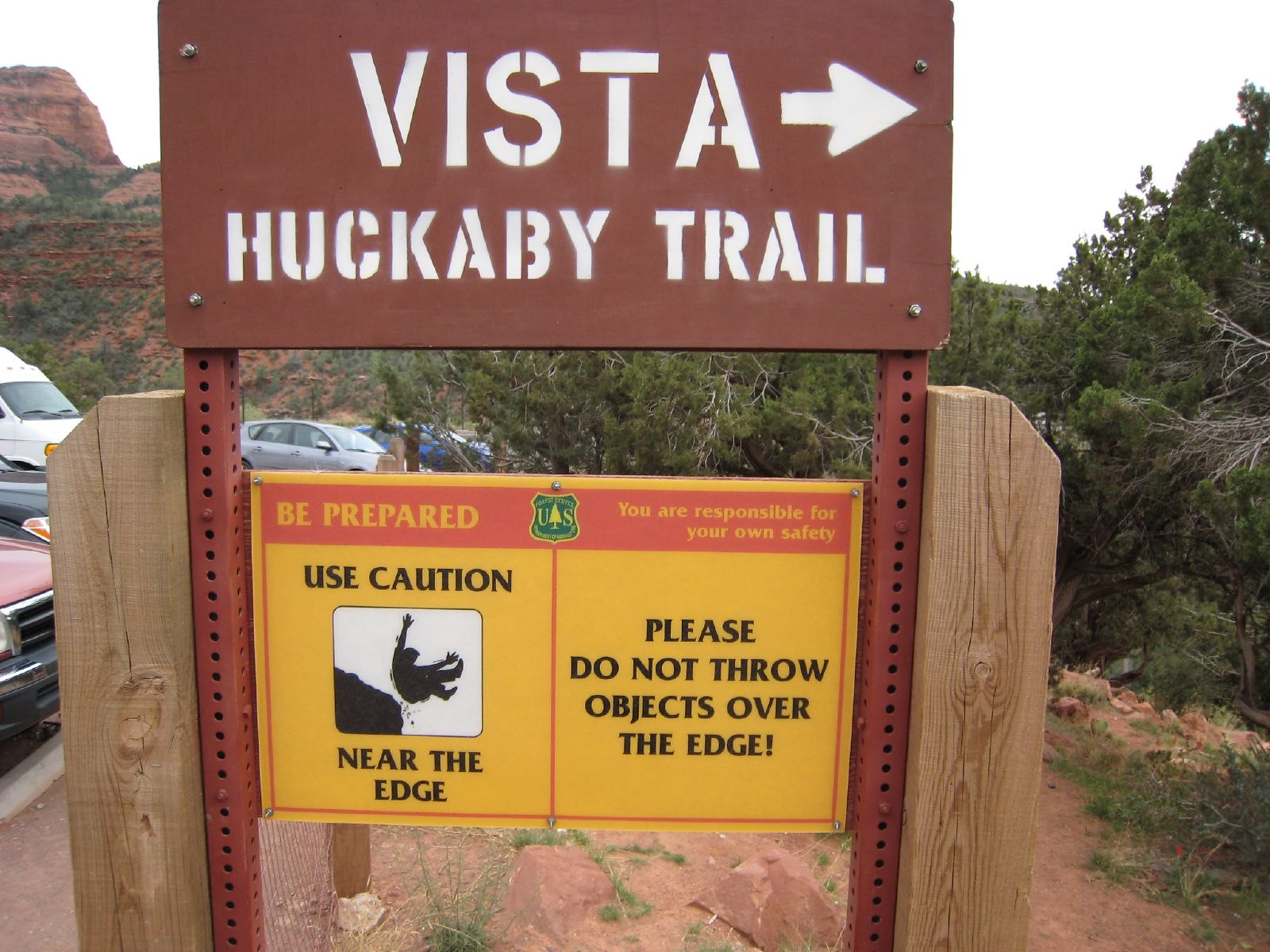The image captures an outdoor setting featuring a prominent, brown wooden sign held up by metal bars and additional wooden supports. The sign, marked with white spray-painted words, reads "Vista Huckabee Trail" with an arrow pointing to the right. Below this is a bold yellow caution sign with a red top edge. Written on this sign are warnings: "Be Prepared," "Use Caution Near the Edge," "You Are Responsible for Your Own Safety," and "Please Do Not Throw Objects Over the Edge," alongside a silhouette of a person falling. The background showcases a scenic view with large stone hills, red mountains blanketed with grass, green leafy trees, and a portion of a parking lot with several cars. The scene suggests the beginning of a potentially hazardous, mountainous trail surrounded by dense woods.